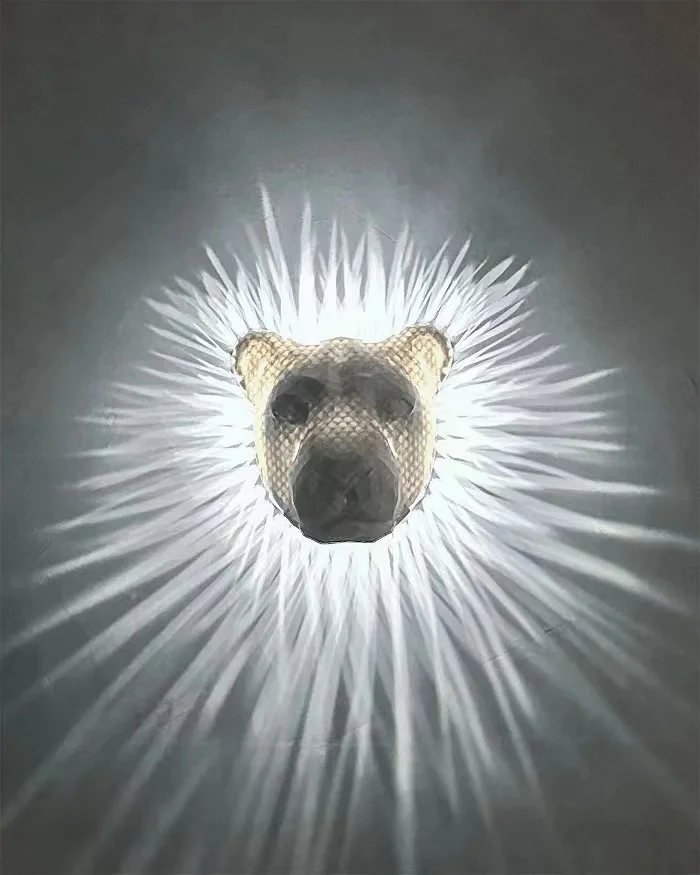This modern digital artwork features the head of a lion cub emerging from a collar of radiating white rays. The lion cub’s face is predominantly a golden yellow with irregular, checkerboard-like markings adding texture to its forehead and cheeks. Its eyes and the area around its nose and mouth are shaded black, providing a stark contrast against the yellowish hues. The cub's short, rounded ears display detailed shading that differentiates the tips from the inner sections. The head appears to be floating, without any trace of a body, set against a dark, gray-green background. The white rays surrounding the head resemble sunrays, emanating outward and creating a bright, almost blinding aura around the creature's face. This unique composition blends elements of abstract imagery with a realistic portrayal of the animal, leaving its exact species open to interpretation, potentially being either a dog or a bear cub.